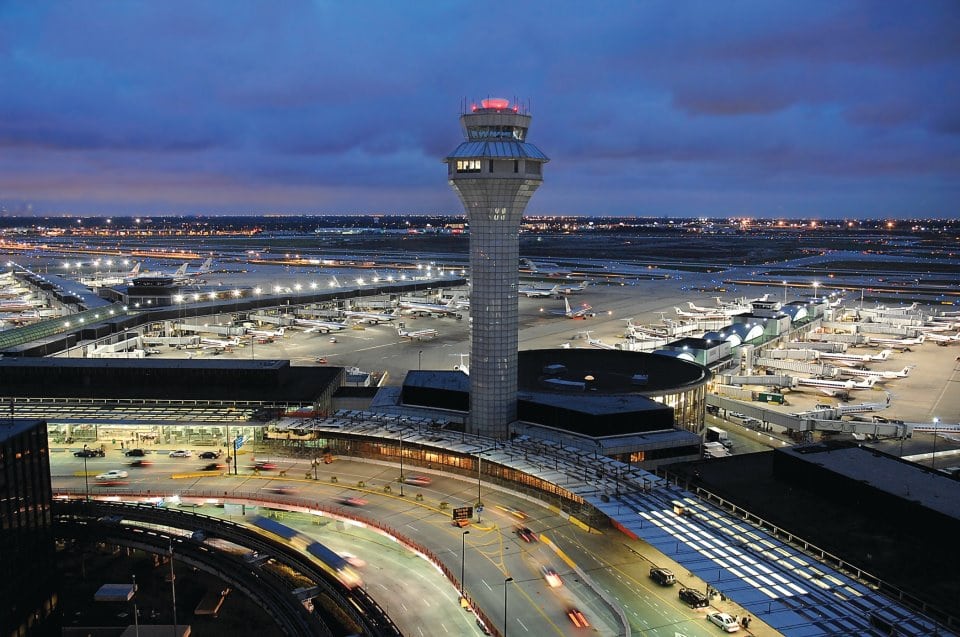This aerial image captures a bustling airport scene dominated by a towering watchtower at its center. The tower boasts a gray facade marked by illuminated yellow square windows and a rounded top adorned with bright orange lights. Above the central circular section, which is gray and framed by five square, yellow-lit windows, the roof transitions from blue to additional gray sections with more windows. The sky behind the tower features a dramatic blend of dark and light blue clouds with hints of orange haze in the bottom left.

The airport itself is a hive of activity, with approximately 20 white airplanes parked on the expansive concrete grounds, though one stands out in blue. The image also showcases a detailed road network at the bottom, with grey asphalt marked by white and yellow lines, curving from the bottom right to the bottom left of the scene. Despite the wide coverage of the airport, city lights are visible in the distant background, adding depth to this atmospheric scene.